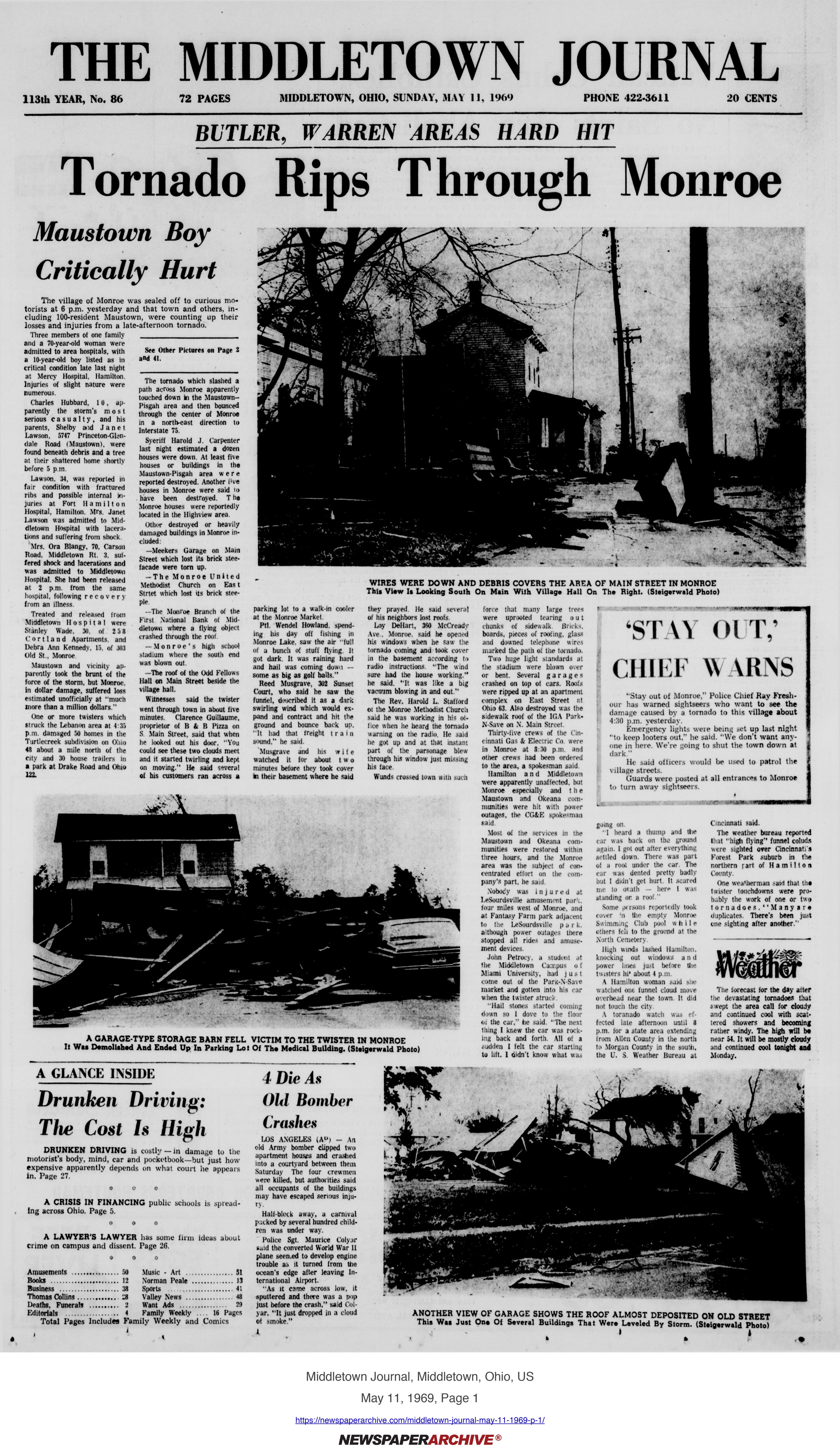This image is a digital scan of the front page of the Middletown Journal, a historic black-and-white newspaper from Middletown, Ohio, dated Sunday, May 11th, 1969. At the top of the page, the newspaper's title "The Middletown Journal" is prominently displayed in a bold, traditional font. Below the title, details including "113th year, number 86, 72 pages," the date, phone number, and price of "20 cents" are provided in a smaller font. The prominent headline reads, "Tornado Rips Through Monroe," underscored by the subtitle "Butler Warren Area's Hard Hit." Adjacent to this headline, in italics, is a sub-headline reading "Moose Town Boy Critically Hurt." The page features three black-and-white photographs depicting the destruction caused by the tornado. The primary image on the right shows a house reduced to wreckage. Another photo on the left, in the middle of the page, captures a building and a car amidst the debris. The third image is more detailed, showing a garage that has nearly lost its roof, labeled with a caption below. The bottom section of the page contains articles with smaller, densely packed text, including a story titled "Drunken Driving, The Cost Is High." The overall layout is filled with numerous articles and detailed reporting, characteristic of a full newspaper page. A notable element at the very bottom right indicates that this is a newspaper archive.